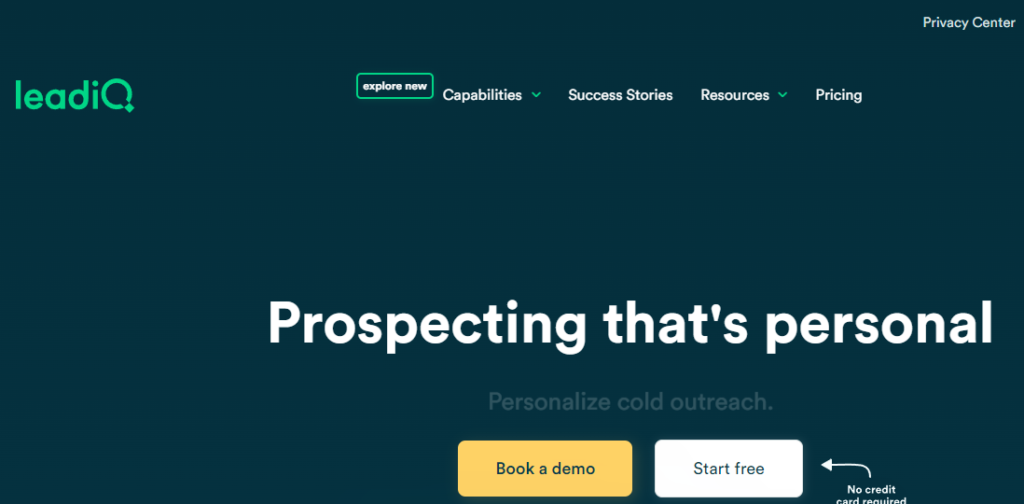In this image, a dark blue background serves as the canvas for a user interface design. Positioned in the top-left corner is the "Lead IQ" logo in green font. Below it, a green-outlined box contains the words "Explore New." 

Adjacent to the "Explore New" box, several navigation options are seen with accompanying down arrows: "Capabilities," "Success Stories," and "Resources," followed by a "Pricing" button without a down arrow. 

In the upper-right corner of the image, the term "Privacy Center" is displayed, likely a clickable link or button.

Dominating the center of the image, large white text reads "Prospecting That's Personal." Below this main headline, a smaller text line describes the feature: "Personalized Cold Outreach."

Towards the bottom, two prominent buttons can be seen: a yellow button labeled "Book a Demo" and a white button labeled "Start Free." Below the white button, there is a note with a small white arrow indicating "No credit card required."

All these elements come together to provide a detailed description of Lead IQ's personalized prospecting features, along with easy-to-navigate options for learning more about capabilities, success stories, resources, and pricing.